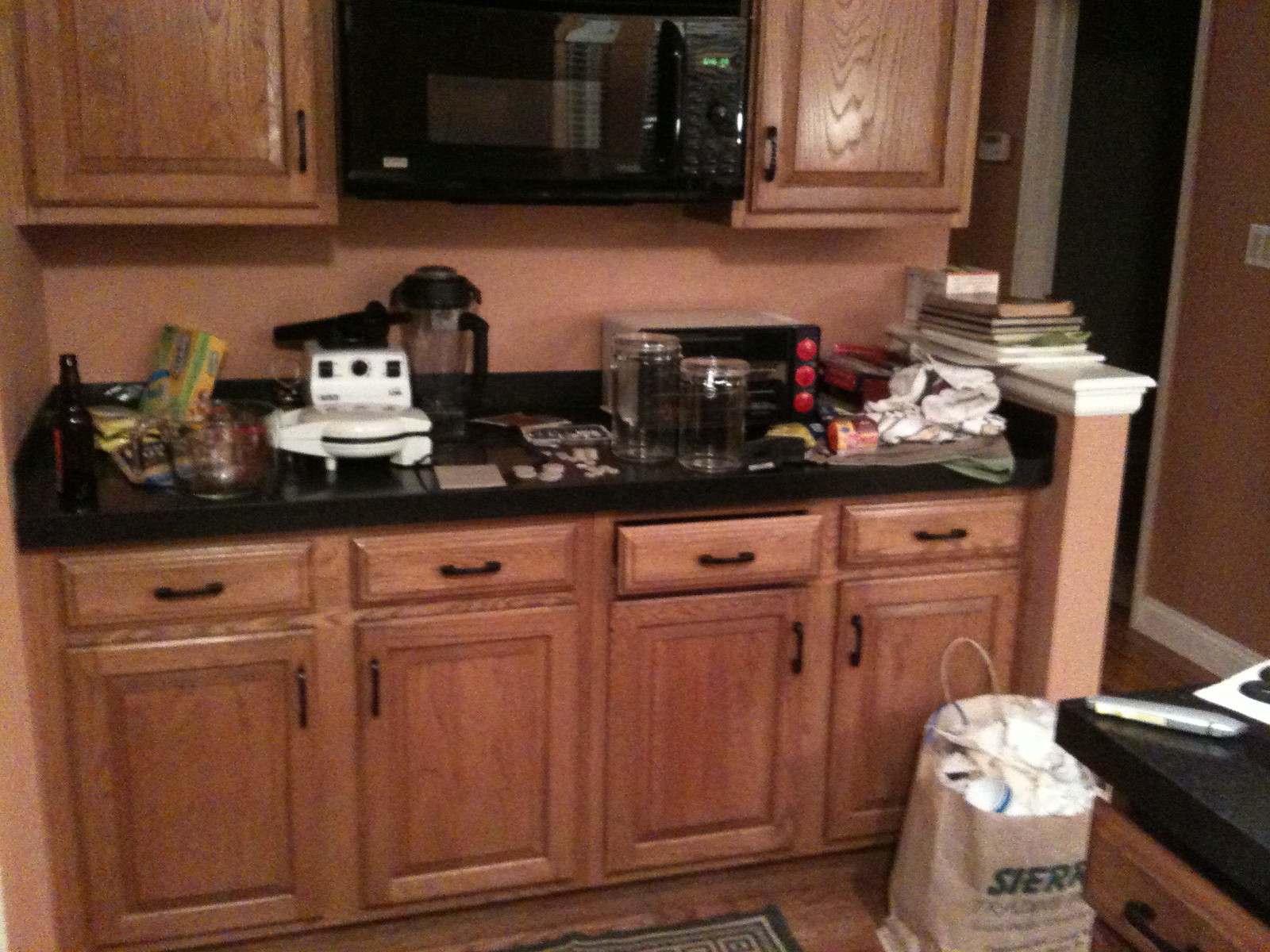The image is a highly detailed photograph capturing the interior of a cozy kitchen. The focus of the scene is predominantly on the left side, characterized by warm, beige walls with a hint of reddish tinge, either due to paint or wallpaper. The left side of the kitchen features an array of brown wooden cabinets—both base and wall-mounted—adding a rustic touch to the room. 

In the center of the cabinetry, a black microwave with faint green text on its digital display is situated, lending a modern contrast to the wooden surroundings. Below the microwave, a black countertop stretches across, cluttered with various kitchen appliances including a white waffle maker, a black juicer, and a distinctive black and gray toaster with red buttons. Additionally, the countertop is adorned with assorted items such as books, green and yellow boxes, and a black bottle.

The cabinetry beneath the countertop includes four wooden units, each featuring a top drawer and spacious storage compartments behind doors. The kitchen floor is made of dark hardwood, and a dark rug is positioned at the center, adding to the homey atmosphere. 

In the foreground, there's a brown paper bag labeled "SIERR" in dark text, which adds a touch of lived-in authenticity to the scene. To the right of the image, there's a hallway with beige walls and white trim, leading to an open doorway into a dimly lit room in the background, providing a sense of depth and space to the composition.